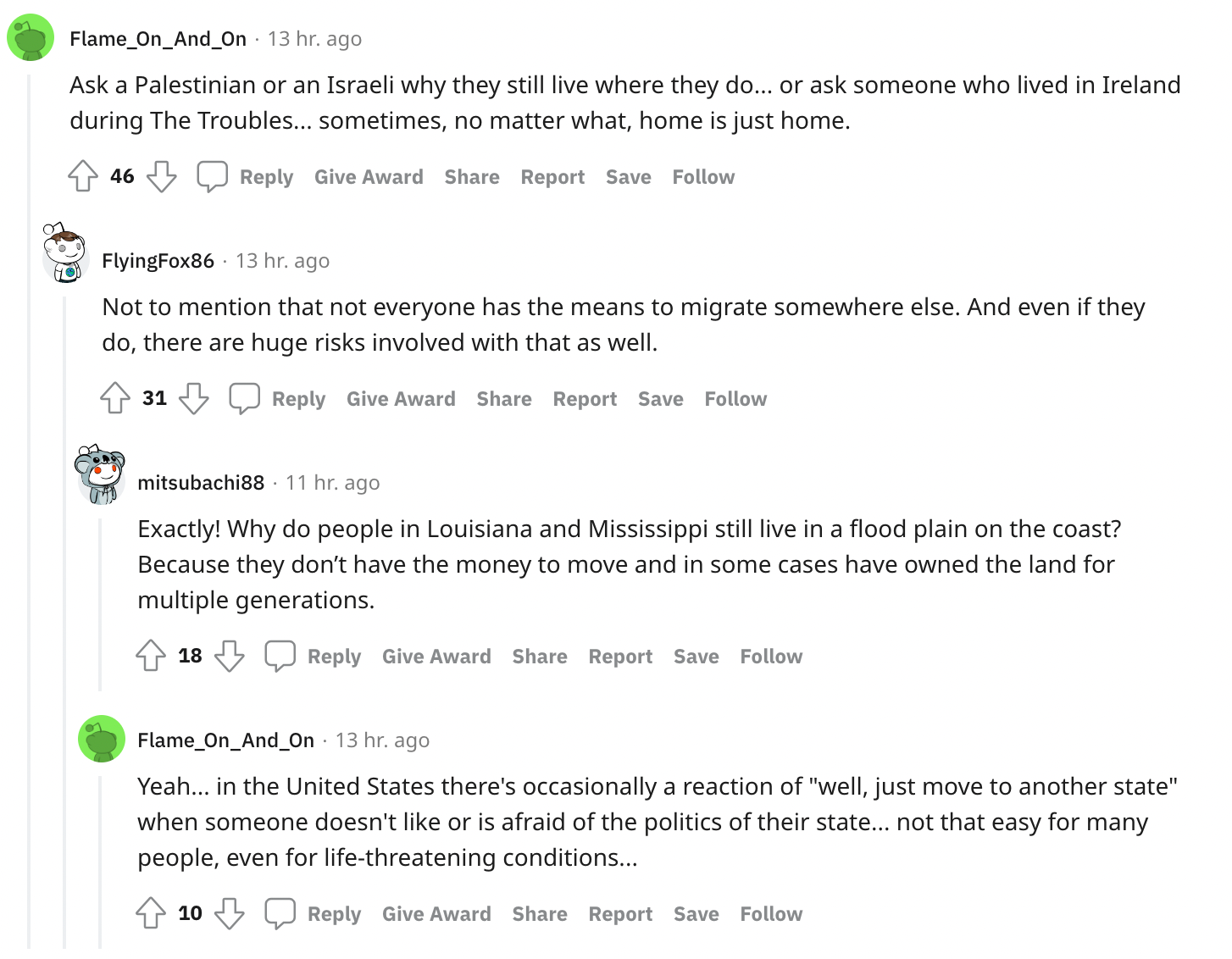This is a detailed screenshot of a comment thread on Reddit, primarily featuring two users engaged in a conversation about the complexities of living in conflict zones. 

The first comment, posted by the user "flame_on_and_on," who has a green default Reddit avatar, is situated at the top. This comment reads: "Ask a Palestinian or an Israeli why they still live where they do... Or ask someone who lived in Ireland during the Troubles... Sometimes, no matter what, home is just home." This comment has garnered 46 upvotes. There are various interaction buttons available beside this post, including upvote, downvote, comment (for replying), as well as options to give an award, share, report, save, and follow.

The subsequent reply is from "FlyingFox86," posted 13 hours ago. This user adds to the discussion by highlighting another critical factor: "Not to mention that not everyone has the means to migrate somewhere else. And even if they do, there are huge risks involved in that as well."

These comments and interactions perfectly encapsulate a poignant discussion on the challenges and emotional ties associated with living in conflict-stricken areas.